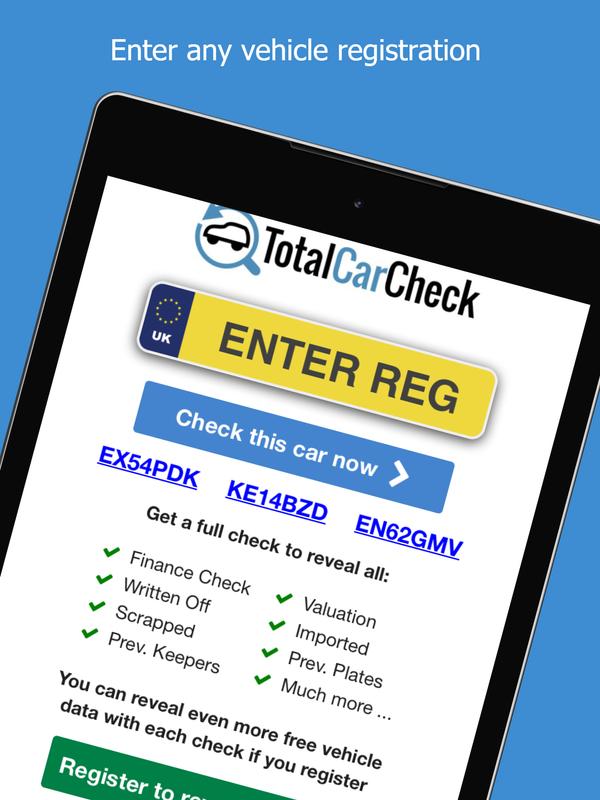The image features a smartphone or tablet screen displaying a webpage for "Total Car Check." The webpage is predominantly themed in a royal blue color. At the top, a black strip frames the page, highlighting the text "Enter any vehicle registration," which stretches across the entire width from left to right. Below that, the "Total Car Check" logo is prominently displayed. The words "Total" and "Check" are in black, while "Car" is in blue. Next to the logo is an icon depicting a car encircled by a magnifying glass with an arrow, symbolizing a comprehensive car inspection.

Towards the middle of the screen, there is a section prompting users to "Enter reg," referring to the vehicle registration number. This section includes a label "UK" on the side. The background here is either black or navy, adorned with white or yellow dots arranged in a circular pattern. The text "Enter reg" is highlighted in yellow.

Further down, there is a blue clickable button labeled "Check this car now," indicating the next step for users. At the very bottom of the screen, a green area features the text "Register to," suggesting an additional registration process.